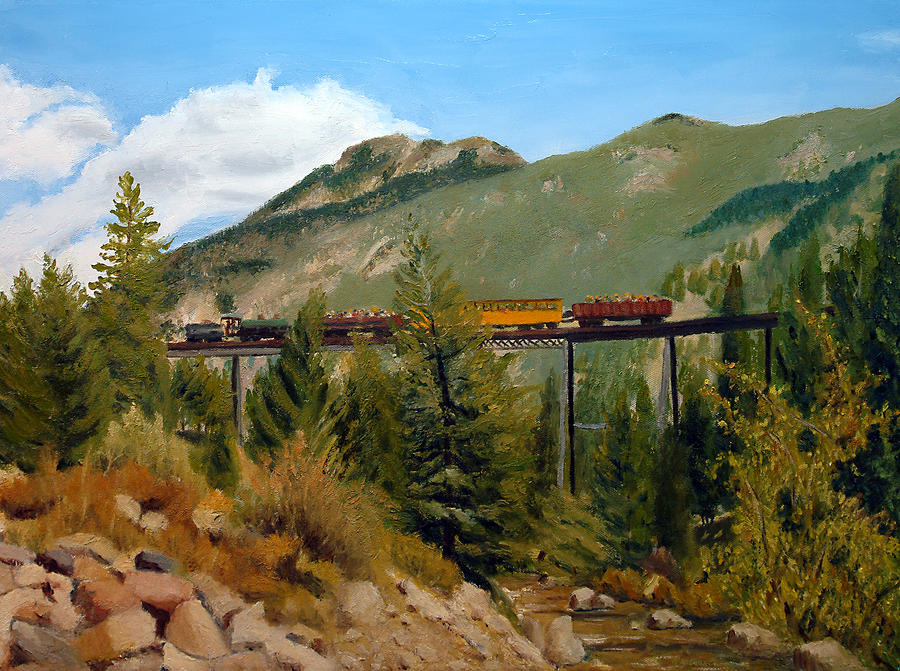The image is a detailed and vibrant painting, possibly an oil or watercolor, capturing a picturesque mountainous landscape. Dominating the scene is an elevated train trestle spanning a deep ravine, which is populated by rugged rocks and a stream. The train, comprising five cars, is painted with a vivid mix of colors: a red caboose, a yellow section, a red car, a green car in the front, and another open car. Some of the cars are open-air and filled with tiny figures, suggesting it might be a tourist train. The background features lush green hills, adorned with dense coniferous trees with occasional yellow foliage. Above, a bright blue sky filled with fluffy white clouds completes the serene outdoor setting. In the foreground, the terrain is rocky, with sporadic patches of grass and foliage enhancing the natural beauty of the scene. The overall atmosphere evokes a sense of tranquility and timelessness, possibly reminiscent of rural landscapes such as West Virginia.